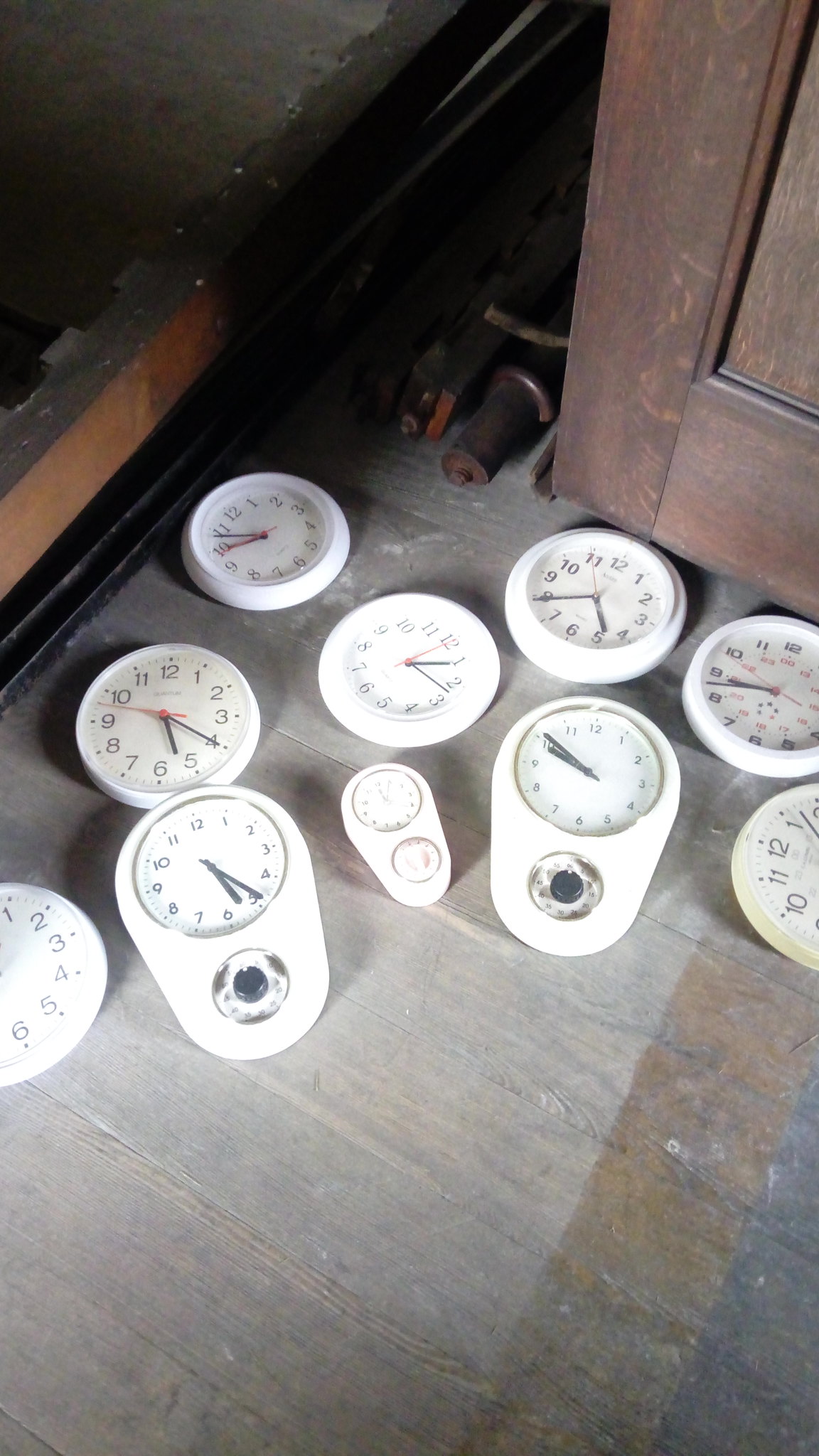The image is a color photograph taken from an aerial viewpoint, capturing a detailed display of various clocks and timepieces arranged on a wooden floor. The wooden floor transitions from light brown to medium brown, then to a dark brown shade. There are a total of ten clocks: seven flat, round, analog clocks with white faces and black numbering, designed to be hung on a wall, and three cylindrical pedestal clocks, each topped with a clock face and appearing to have a light fixture. The clocks are meticulously placed in an east-west direction in the middle of the floor. Behind the arrangement, there is medium brown cabinetry visible, suggesting a cupboard in the background. The clocks vary in size, with some featuring dual clock faces while others have a single face, all equipped with minute, second, and hour hands, meticulously presenting the intricate details of their designs.